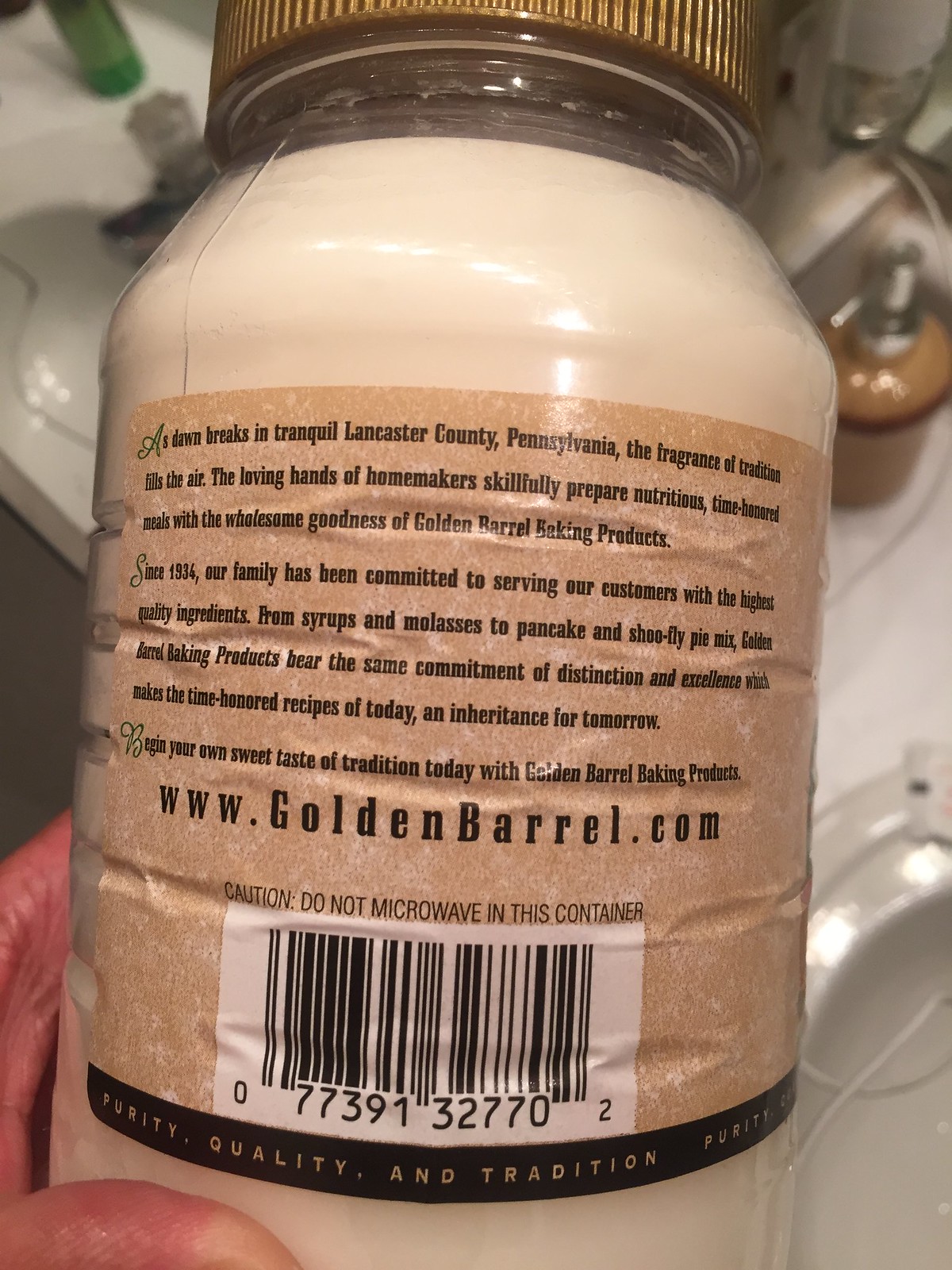In this color photograph, a person's hand is visible in the bottom left corner, firmly holding a glass jar. The jar is capped with a ribbed, gold-colored lid that adds a touch of elegance to the rustic contents within. The back label of the jar is prominently displayed, adorned with intricate text that reads: "As dawn breaks in tranquil Lancaster County, Pennsylvania, the fragrance of tradition fills the air. The loving hands of homemakers skillfully prepare nutritious, time-honored meals with the wholesome goodness of Golden Barrel Baking Products. Since 1934, our family has been committed to serving our customers with the highest quality ingredients. From syrups and molasses to pancake and shoofly pie mix, Golden Barrel Baking Products bear the same commitment of distinction and excellence, making the time-honored recipes of today an inheritance for tomorrow. Begin your own sweet taste of tradition today with Golden Barrel Baking Products. Caution, do not microwave in this container." A barcode numbered 077391327702 sits close to the bottom of the label. Further enhancing its heritage feel, a black banner at the base of the label proudly proclaims, "Purity, Quality, and Tradition."